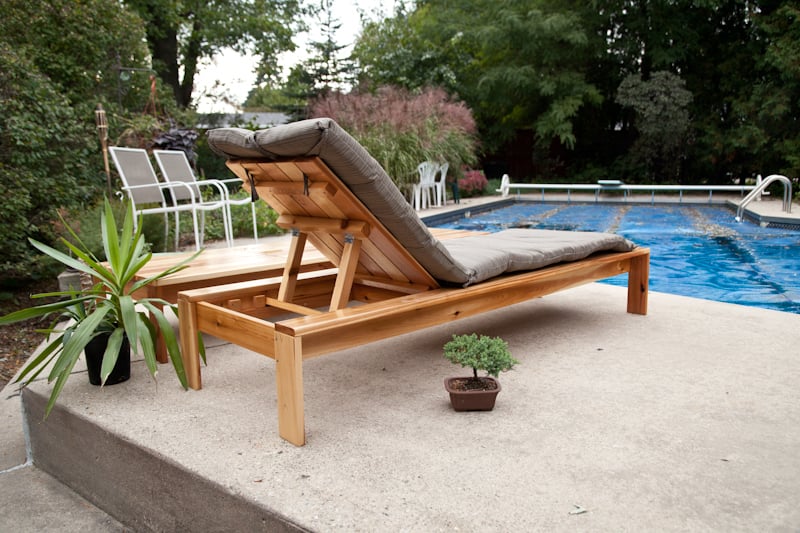The photo is taken outdoors and captures a serene swimming pool scene. The pool, which has bright blue water and three lanes, is located in the right center of the image. On the right side of the pool, there's a metal ladder leading into the water, and a diving board is visible at the back middle section of the pool. The pool area is surrounded by a lush landscape, including a thick forest of trees in the background and tall shrubs with purple blooming tops in the left corner.

In the foreground, there is a concrete base that supports a wooden lounge chair with a gray cushion, positioned upright and facing the pool. Adjacent to the lounge chair on the right is a small green bonsai plant, and to the left, a larger green leafy plant sits in a black pot. The surface they rest on is beige and has a rough texture. Additionally, white metal chairs are arranged along the left side of the pool, extending towards the back. The area has a peaceful ambiance, enhanced by the natural greenery surrounding the pool and the organized seating arrangement that invites relaxation.